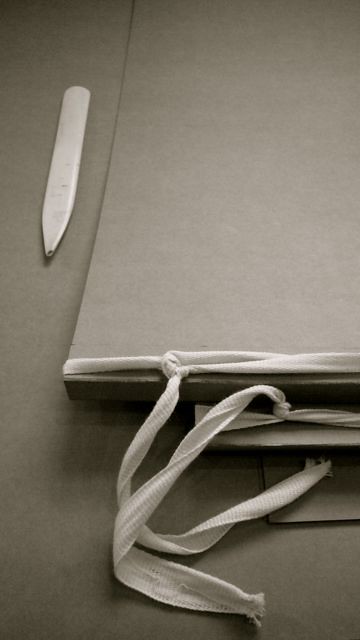The photograph depicts a grayscale image of a rectangular, vertically-oriented object that could be a bag or a board with string tied around its top. The entire scene is rendered in shades of gray, consistent with a black-and-white photograph. The main object is gray and appears to have a white, cloth-like string wrapped around its upper part, tied into a knot. Below this, another section of the object also features a smaller white string tied similarly. This object might contain a dark, rectangular, hard item visible at the top. Adjacent to this object, positioned towards the top left corner of the image, is a white, flat, pencil-like object. It has a pointed end at the bottom, suggesting it could be a writing instrument or a similar tool. The entire setup rests on a gray, flat surface, possibly a table or counter. There is no text, date, name, or people visible in the photograph.